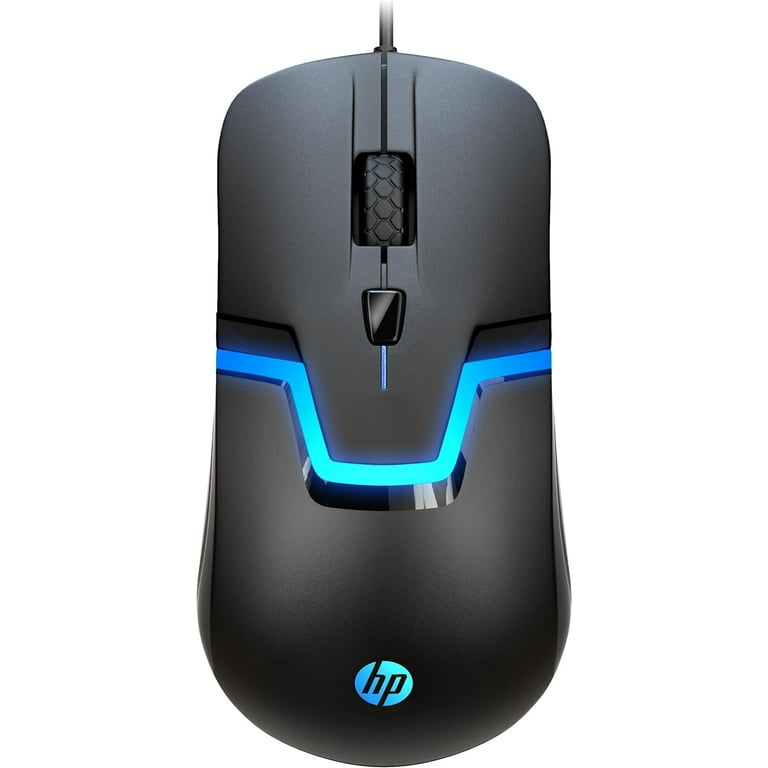This is a close-up image of a black HP computer mouse against a completely white background. The mouse is wired, with the black cord extending from the top, though the cord is partially cut off in the image. The mouse features a neon blue U-shaped light design in the middle, which runs just below a scroll wheel (referred to as a tread or thumb wheel) and a button situated under this scroll wheel. The HP logo is positioned at the bottom of the mouse, illuminated in a light blue color. The body of the mouse tapers slightly toward the wired end and has a bulbous shape at the other end. There are no side buttons visible in this image.